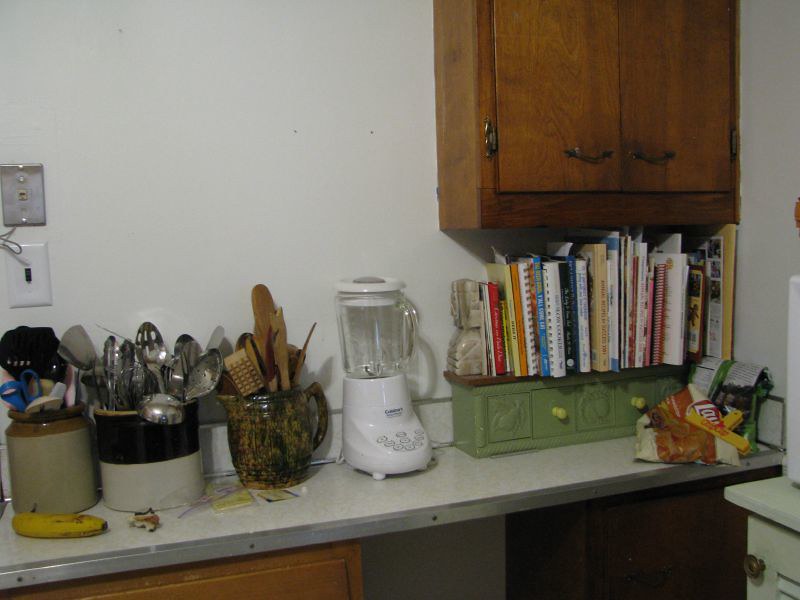The image depicts a vintage kitchen countertop made of white faux marble laminate with a metal trim secured by nails along its edge. On the right side beneath the counter is a dark cabinet, while on the left bottom, an oak-colored cabinet is visible. 

The countertop is adorned with an array of kitchen items, starting from the left. First, there is a clay pot holding various kitchen utensils, including a blue-handled pair of scissors, spoons, and spatulas. In front of this container lies a very ripe banana. 

Next to it is a container brimming with silver kitchen utensils, featuring straining spoons, tongs, and spatulas, all metallic. Adjacent to this is a charming clay pitcher with a handle and spout, filled with wooden utensils. 

Further along, there is a white and clear glass blender. Finally, a small green shelf teeming with old cookbooks is positioned at the right end of the countertop.